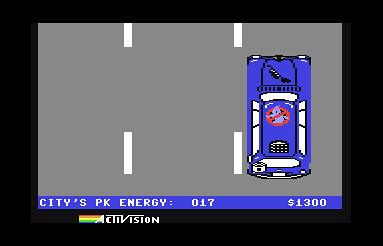The image depicts a bird's-eye view of an old video game screen bordered by a black frame. Central to the image is a gray road sectioned by white dashed lines, resembling highway markings. The focal point is a blue car featuring the iconic Ghostbusters logo—a ghost within a red circle, crossed by a red line—on its roof. The car has white windows on all sides. Below the car, a blue banner with white text reads "City's PK Energy -- 017" and displays a money amount of $1300. At the very bottom, "City Vision" is presented in vibrant lime green, yellow, and orange letters. Additionally, there is a rainbow-striped logo beside the gold-lettered "Activision," suggesting the game developer's name.